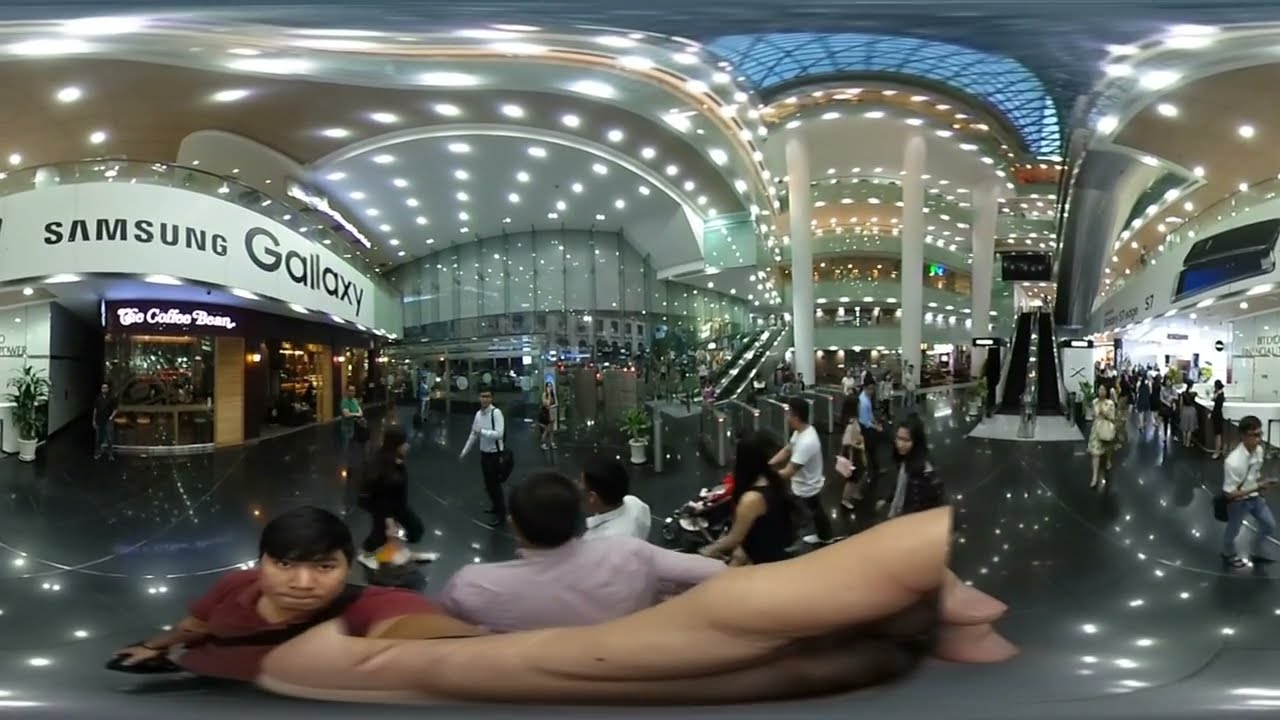The panoramic 360-degree image captures the bustling interior of an expansive open corridor within a shopping mall, distinguished by an extremely high vaulted ceiling. The scene is filled with bright white lights reflecting off various surfaces, illuminating the space vividly. On the left, one wall features a prominent Samsung Galaxy marquee, styled with the recognizable Samsung font, and directly beneath it, a smaller sign for "The Coffee Bean" in a cursive, italicized font. Tall white pillars reach up towards the ceiling, and behind them, several different stories of the mall are visible, each fronting the same open courtyard below.

The foreground is populated with numerous people, particularly notable is an indeterminate-gender Asian individual in a red short-sleeved top. This person's arm appears highly distorted due to the curvature introduced by the 360-degree lens, as they seemingly reach out towards the camera, possibly taking a selfie. Adjacent areas include additional shops and a wall of windows or glass, enhancing the feeling of openness and multi-level complexity. Small details such as an 'S7' branding on the right and milling crowds further accentuate the lively and dynamic atmosphere of this commercial space.